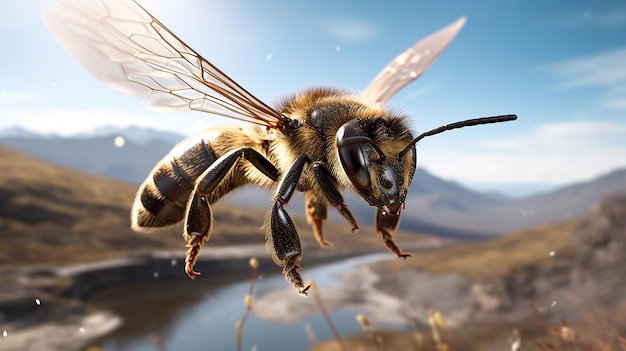This image features a close-up of a honey bee, rendered in stunning 3D detail. The bee appears to be suspended midair, flying from the left side of the screen towards the right, with its semi-transparent, slightly colorized wings showing no signs of movement, giving it an almost floating appearance. The bee is characterized by its fuzzy yellow and black fur, black legs extending outward, and black antennas and eyes. In the backdrop, a blurry stream flows through a valley with pollen floating in the air. Majestic mountains can be seen in the distance under a clear blue sky dotted with white clouds, adding to the depth and realism of the scene. This intricate capture, possibly from a drone due to its elevated perspective, highlights every detail of the bee, from its burly body and thick legs to its potential for a gnarly sting.